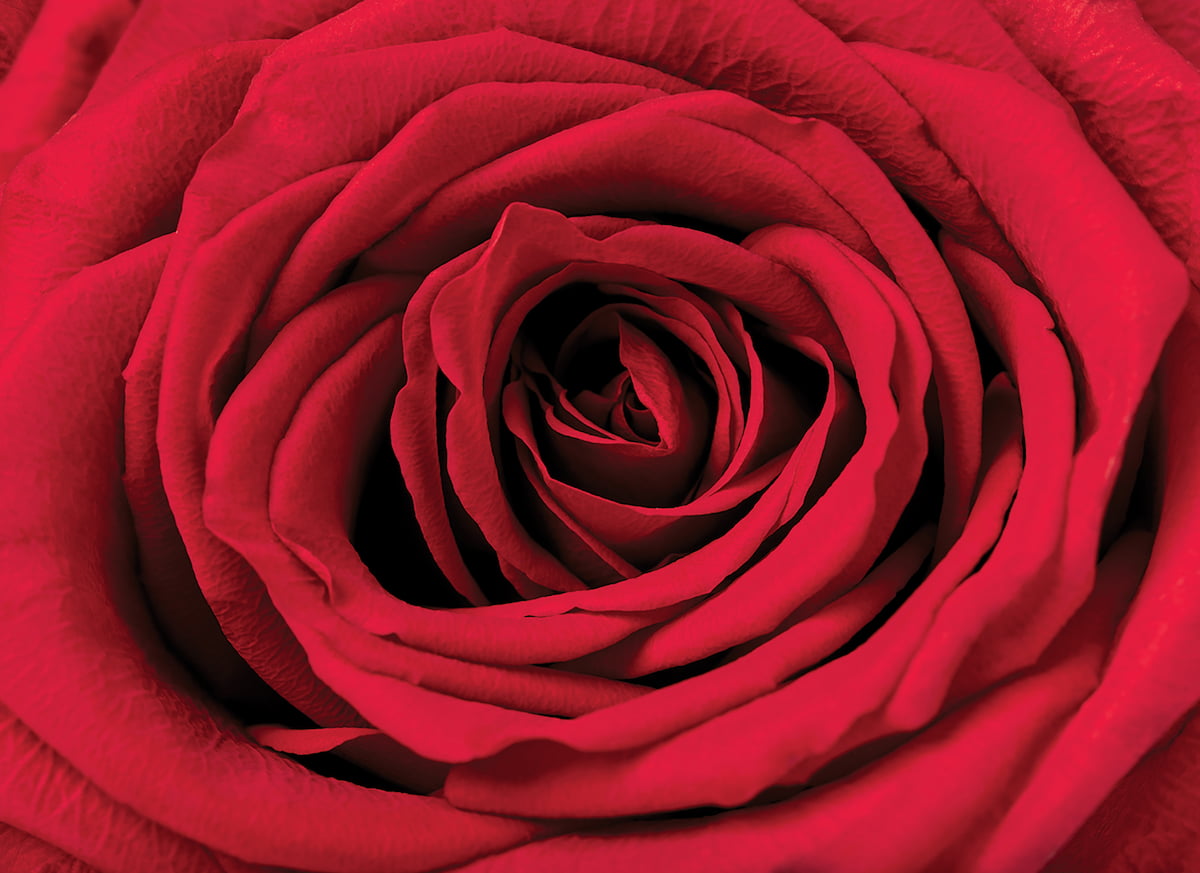This image captures a stunning, close-up view of a single, vibrant red rose. The focus is entirely on the intricate petals, which appear to spiral inward, creating an almost hypnotic effect. The petals are layered closely together, starting tightly in the center and gradually expanding outward, reminiscent of a beautifully crafted paper mache. The high-resolution photograph reveals an astonishing amount of texture and detail, highlighting the deep shadows between the petals and making the red hue the dominant feature of the image. The rose looks exceptionally healthy, with no visible wilting or damage, and the overall composition fills the entire frame with rich, even red, punctuated by subtle dark shadows.